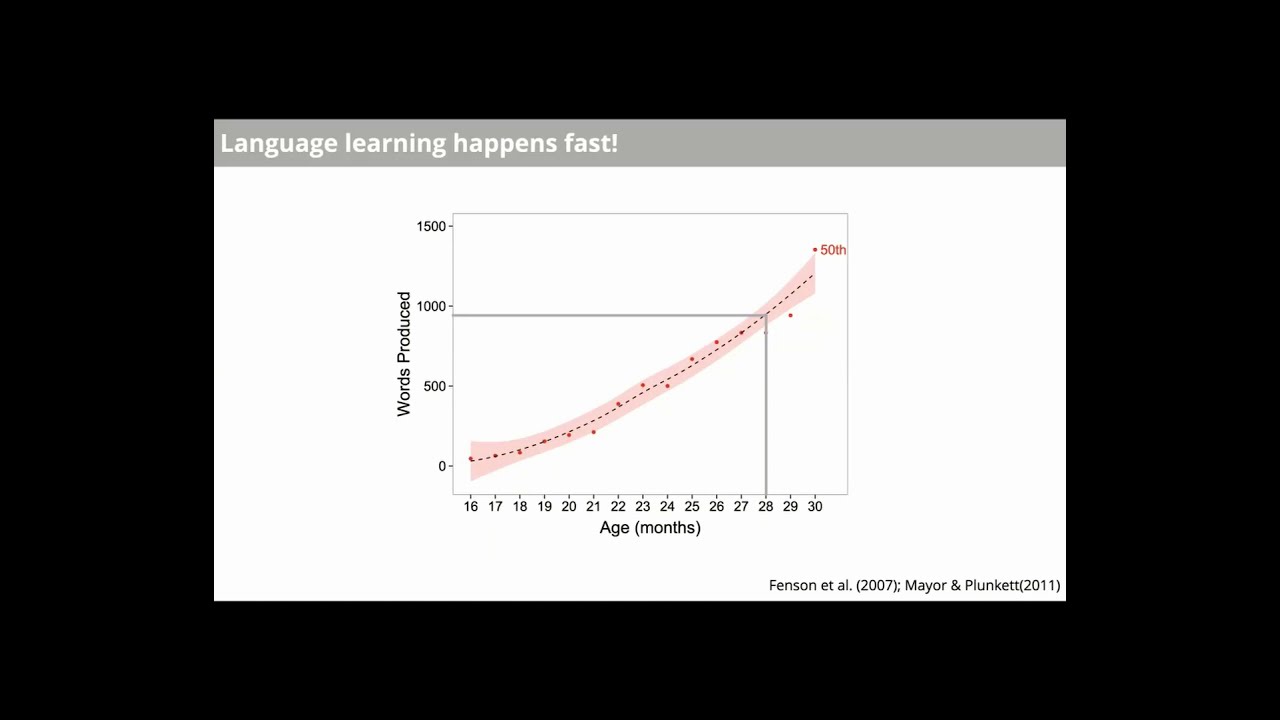The image features a computer-generated line chart set against a white background within a larger black rectangle. At the top center, a gray border with white text reads, "Language learning happens fast!" Below this, a graph dominates the white rectangle. The vertical y-axis is labeled "Words Produced," ranging from 0 to 1500, while the horizontal x-axis is labeled "Age (months)," spanning from 16 to 30 months. The graph showcases a curved, dotted line that starts at the left edge and rises steeply towards the right, almost reaching the top. Small dots punctuate the line, suggesting data points. A gray line aligns just under the 100-mark on the y-axis, extending horizontally before descending vertically to the 28-month mark at the bottom. In the bottom right corner of the white rectangle, a citation reads "Fenson et al., 2007. Major and Plunkett, 2011."